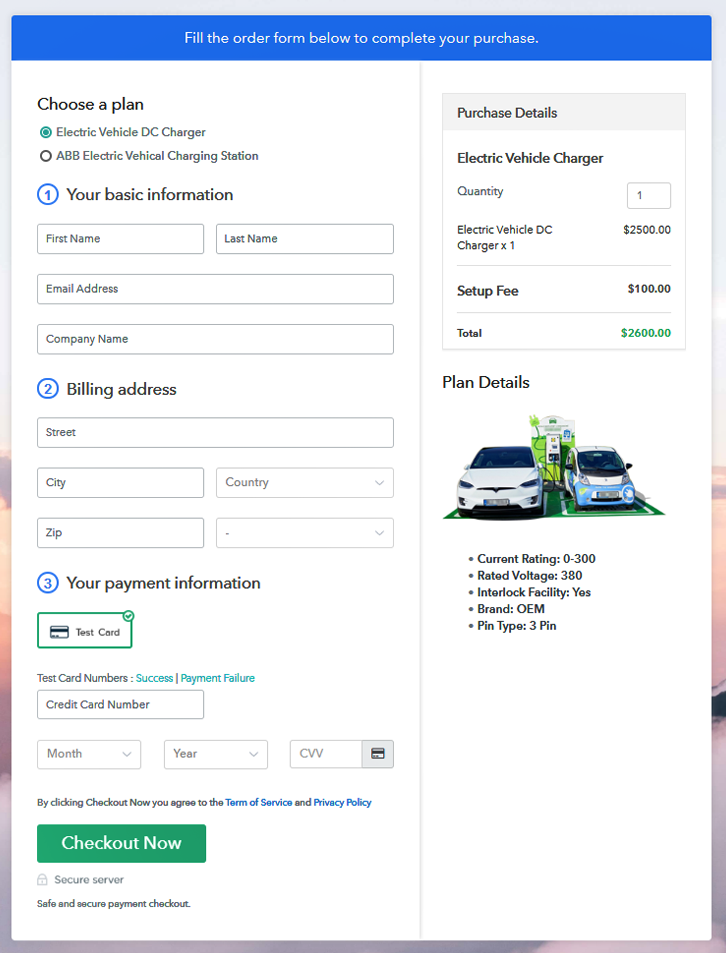This is an image of a website interface, featuring a prominent header and sidebar layout. The top section of the page, as well as sections halfway down on the left and right sides, are shaded in gray. Just below the gray section on the right-hand side, there is a small tab overlapping the image, which is partially visible and appears red. Gray fills the area down to the bottom edge and across the bottom, while extending halfway up the right side where the red tab is.

At the top center of the page, there is a blue border about half an inch wide. Inside the blue border, white text reads, "Fill the order from below to complete your purchase." Below this, the background is predominantly white. About two-thirds of the way across the page, a vertical gray line divides the left section from the right.

In the upper left corner, the phrase "Choose your plan" is displayed in black. Below this heading, a small green circle is labeled "Electric Vehicle DC Charger." Following this, an outlined white circle with black text features "ABB Electric Vehicle Charging Station." Another white circle with a blue border and interior text indicates "Your basic information," with fields for first name, last name, email address, and company name.

Below the personal information section, another blue-bordered white circle is labeled "Billing address," with input fields for street, city, county, and zip code. Further down, under the "Your payment information" section, a green checkout tab is positioned at the bottom left, featuring white text that reads "Checkout." Adjacent to this, the phrase "Secure server" is shown alongside a small lock icon. Below this, the message "Safe and secure payment checkout" is presented.

On the right side of the dividing line, there is a light blue tab with the text "Purchase Details." Underneath, detailed information about the car is displayed.